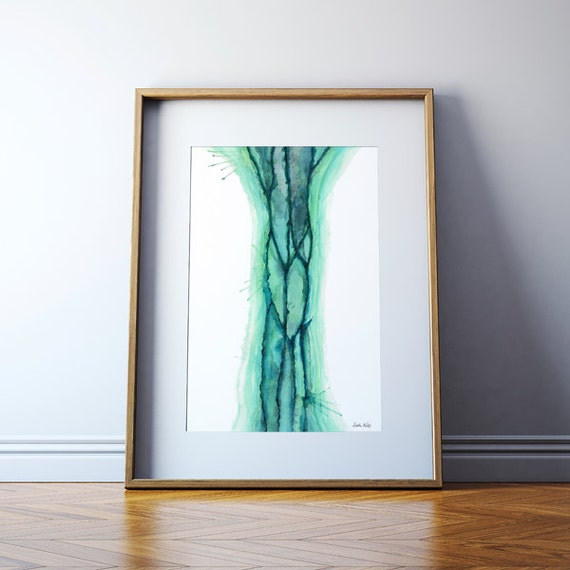The image depicts a rectangular, framed watercolor print leaning against a white wall with a white skirting board. The floor beneath is a tan, brownish parquet wood that reflects the painting slightly. The frame is a light-colored wood, with a thin gold-like trim surrounding a white border. The artwork itself features an abstract design resembling a tree trunk, painted in vibrant turquoise and green tones, with darker green, artery-like lines running vertically from top to bottom. A signature is visible in the bottom right corner of the print, though it is too small to be legible.